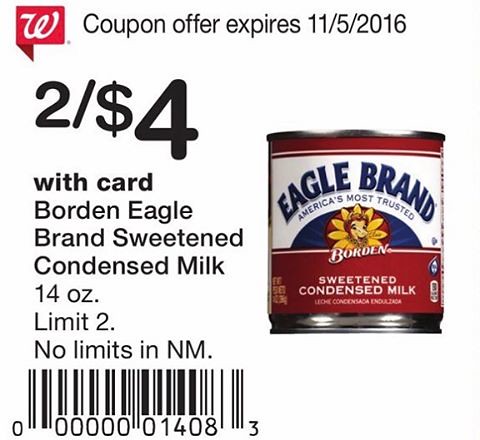**Coupon Description:**

The image showcases a coupon against a completely white background. At the top of the coupon, there is a red rectangle featuring a stylized white "W." Immediately following this in black text, it reads, "Coupon Offer Expires 11/5/2016." Below it, in larger text, it states, "$2/4 dollars," with the dollar sign and number "4" prominently displayed. Further down, it clarifies in black text, "With card Borden Eagle Brand Sweetened Condensed Milk 14 oz, Limit 2 (No limits in NM)." Towards the bottom of the coupon, there is a barcode with the number "000001408" beside it. To the right of the barcode, a small cylindrical can is depicted. The can has silver bands at the top and bottom, with a red label featuring a white band near the top. In big bold blue letters, the label reads "Eagle Brand," followed by "America's Most Trusted" in smaller print. In a blue semicircle, there is an image of a yellow cow surrounded by yellow petals. Below this image, within the red band of the label, white lettering spells out "Borden" and "Sweetened Condensed Milk.”